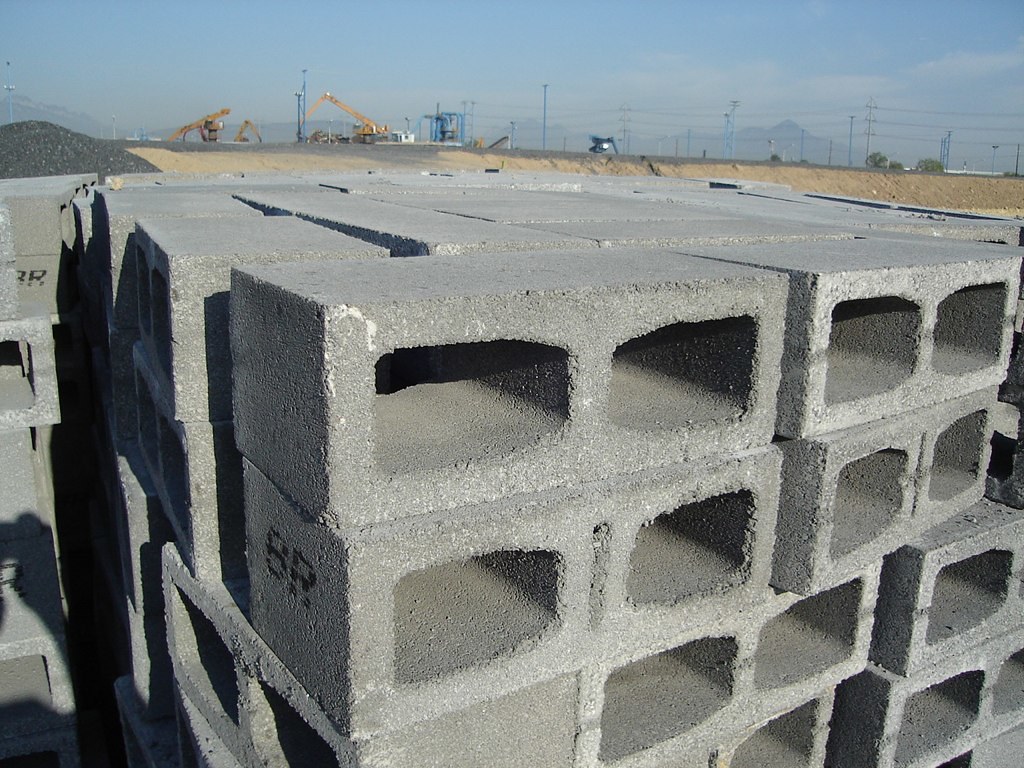In this outdoor photograph, a detailed construction site comes into view. Central to the image is a sizable pile of large, gray concrete slabs stacked approximately seven blocks high and eight to ten blocks wide. Surrounding these slabs, the scene features an array of construction elements including cranes, machinery, and additional materials like what appears to be a coal pile. The foreground contains brown dirt or sand, while scattered trees or bushes dot the periphery. In the distance, a mountainous horizon rises, augmented by visible power lines and electric poles stretching across the landscape. The sky above is tinged with a slight smog, yet retains a light blue color with patches of big, white, fluffy clouds. Additionally, one of the concrete blocks bears the visible symbol "BR." The machinery and cranes, prominently orange, underscore the site's active construction focus. The overall atmosphere suggests a bustling construction zone set against a backdrop of natural elements.